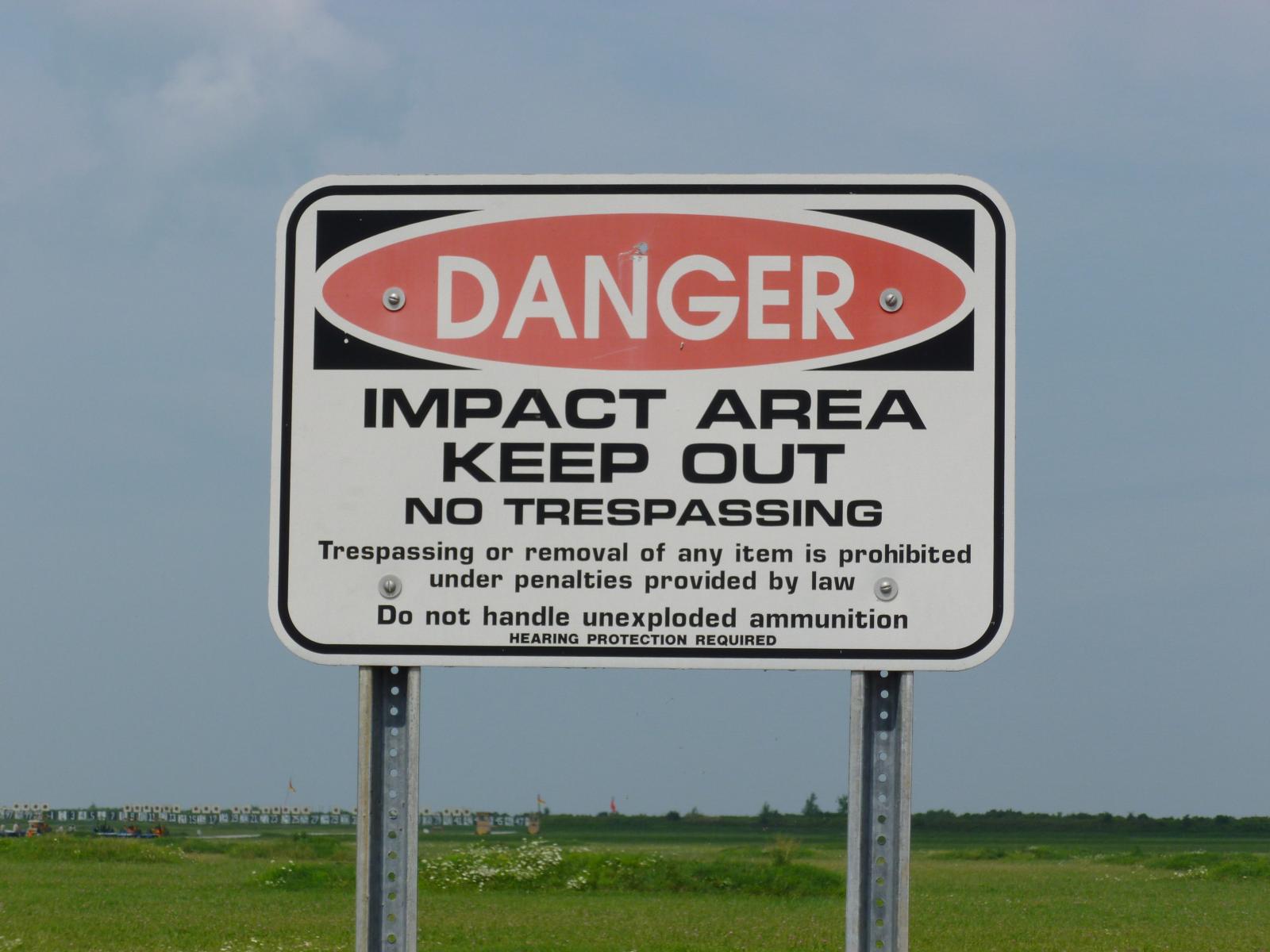In this large, square photo, the background showcases a cloudy sky, predominantly dark bluish-gray, with clusters of white and gray clouds in the upper left-hand corner. At the bottom left of the image, you can spot a distant bridge, presumably arching over some unseen body of water, and the rest of the background is filled with vast fields of grass peppered with white flowers and sporadic trees stretching towards the horizon.

Dominating the foreground are two sturdy metal poles supporting a large, horizontally aligned rectangular sign with rounded corners. This sign has a prominent white background, encircled by a black border. At the top of the sign, a distinctive red oval outlined in white frames the word "DANGER" written in bold, white capital letters. Beneath this red oval, larger black capital letters declare: "IMPACT AREA, KEEP OUT, NO TRESPASSING." In the smaller text below, the sign sternly warns: "TRESPASSING OR REMOVAL OF ANY ITEM IS PROHIBITED UNDER PENALTIES PROVIDED BY LAW. DO NOT HANDLE UNEXPLODED AMMUNITION. HEARING PROTECTION REQUIRED." This suggests a hazardous area, possibly linked to unexploded ammunition, reinforcing the importance of the warning.